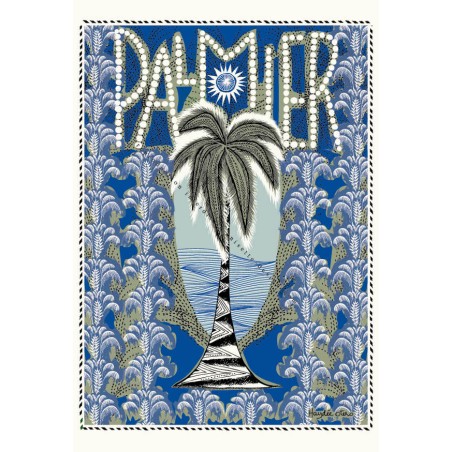This detailed illustration depicts a central palm tree with a black and white trunk featuring white triangles pointing to the right. The extended, dark gray leaves of the palm tree reach approximately halfway down its trunk. The artwork is set against a backdrop of a blue hue decorated with ornate blue flowers arranged in four vertical rows. The image resembles a postage stamp, bordered with a black, rope-like dotted line. At the top of the artwork, the word "PALMIER" is prominently displayed in a font created from white beads or lights, set against a pale green, olive-colored background. Below the "M" in "PALMIER" is a blue orb with a white star-like pattern. The background also includes elements suggestive of water or ocean waves, contributing to the scenery behind the palm tree, which gives the illustration a coastal or tropical feel.